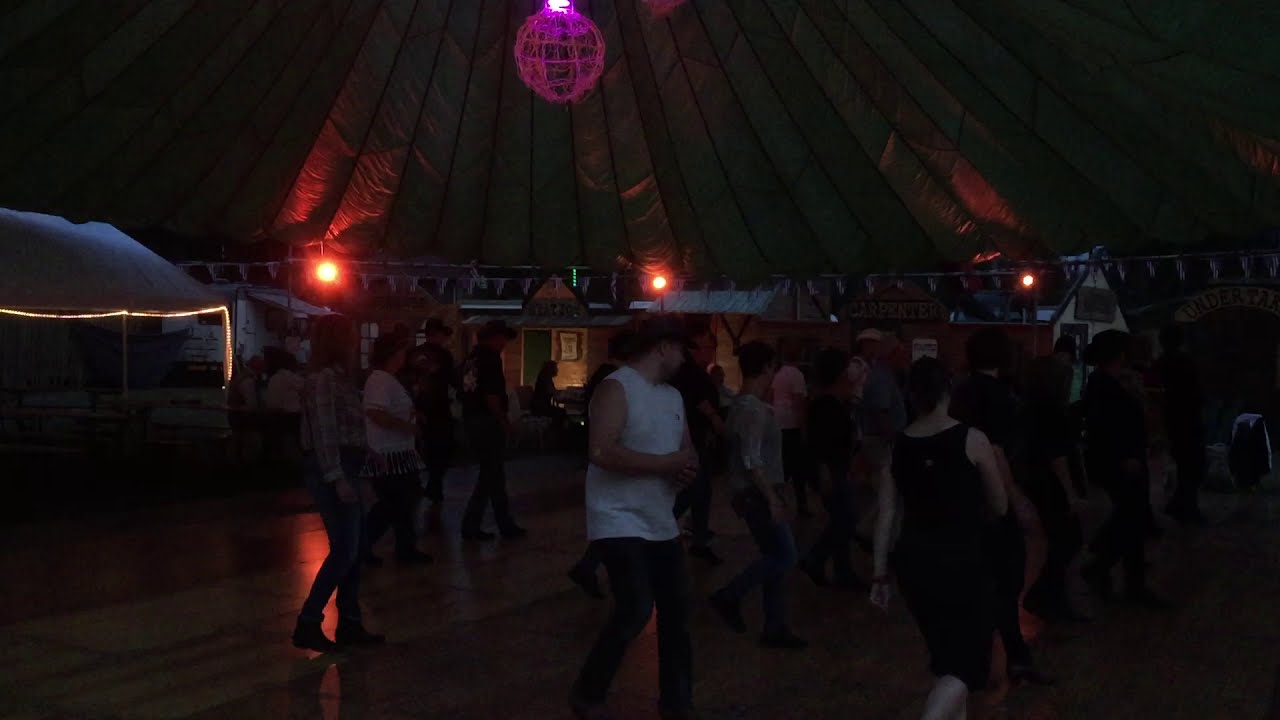In this lively and vibrant photograph, a large group of around 20 to 25 people are enthusiastically engaged in country line dancing inside what appears to be a tented pavilion or a similarly decorated indoor space. The dimly lit environment is illuminated by a pink disco ball-like light fixture hanging from the center of the tent roof, casting a festive glow over the scene. The dancers are dressed in typical country western attire, with lots of blue jeans, cowboy hats, and sleeveless shirts visible. Especially prominent in the middle of the image is a man wearing a loose-fitting white tank top, blue jeans, and a dark cowboy hat. He stands out among the dancers who are all mostly in line formation. To the left side of the image, a white awning adorned with string lights adds to the decorative ambiance. In the background, a white fence with glowing yellow lights and an Alpine-style house can be seen, contributing to the overall festive setting of this celebration.